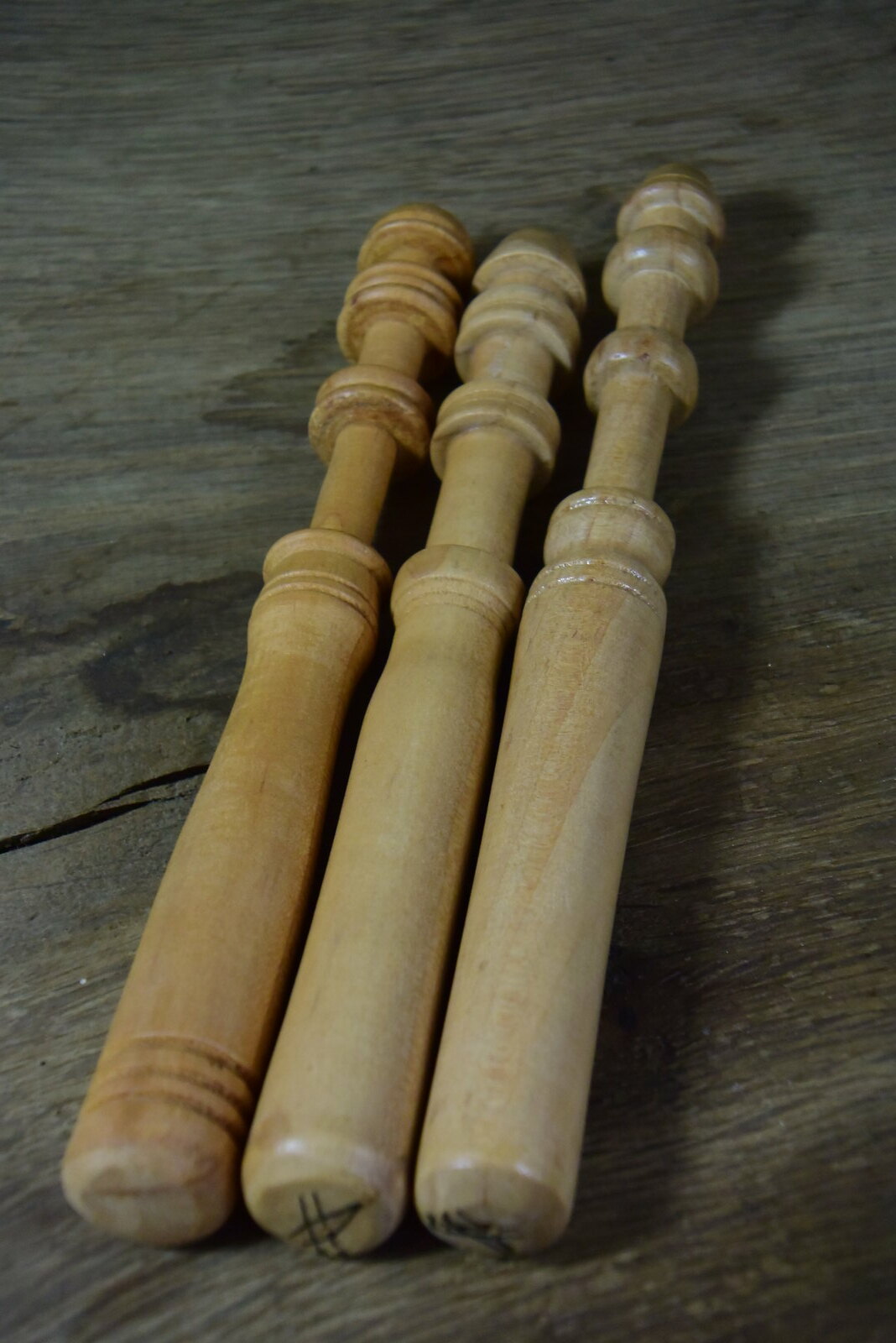In this image, there is a dark gray, unfinished wooden table with noticeable wood grain and a crack in the lower left corner, adding an element of texture. Resting on the table are three intricately carved wooden dowels, likely components of stairway posts, each varying slightly in color and design. The dowel on the far left is a slightly darker, reddish-brown wood, featuring ridges at both the bottom and top. The middle and right dowels are lighter, blond-colored wood, with rounded edges and circular ridges. Each dowel is thick at the base, tapering at intervals created by the circular carvings, ending in round tops. The middle dowel also has a black mark in the shape of a number sign at the top, adding a unique identifier. The detailed craftsmanship and varying wood tones provide a rich visual contrast against the dark background.